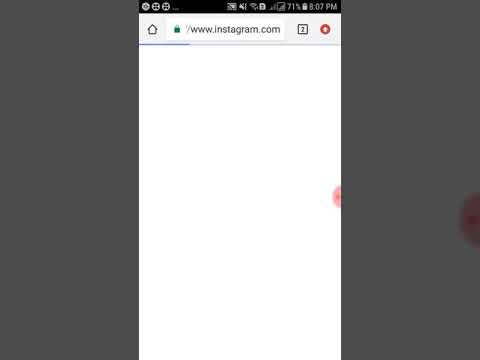The image features a central screenshot from a phone, bordered by gray areas on both the left and right sides. In the right gray margin, there is a noticeable purple spot. This spot also appears in the white area, characterized by a light hue around the edges and darker tones in the center. The top section of the screenshot includes a black bar displaying a 71% battery indicator, the time "8:07 p.m.", and several indistinct icons on the left that are too blurry to identify.

Below this, on the left side, is a home icon. Adjacent to it, the URL bar shows a green lock icon next to "www.instagram.com." To the right of this, there's a square icon that appears to have the number "2" within it. Further to the right is a red, oval-shaped icon that might have an upward arrow, though the image quality makes it challenging to clearly determine.